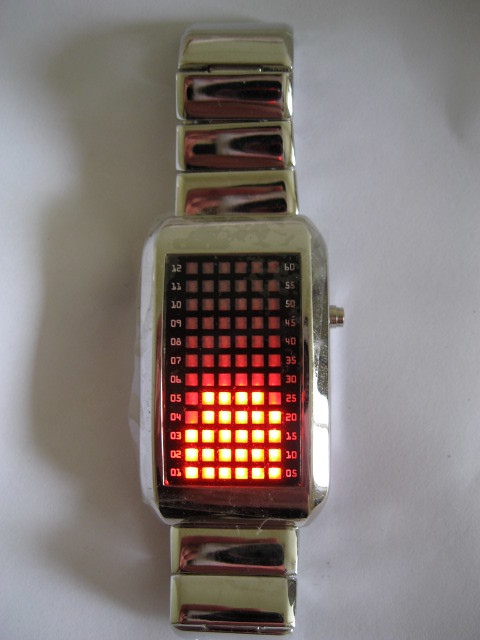A device resembling an Apple Watch, possibly a thermostat, is mounted on a white wall. The device features a sleek silver frame and a distinctive design reminiscent of polished marble, with a pattern of black, light brown, and white running down its center. The front of the device is marked with numbers ranging from 1 to 12 on each side, interspersed with several red dots. Notably, the numbers 4, 20, 5, and 25 each appear to have a missing dot, suggesting some form of selective indicator or calendar. The device's modern aesthetic is complemented by its seamless integration with the wall, highlighting both functional and decorative elements. Shadows cast around it enhance its three-dimensional appearance and confirm it is wall-mounted.